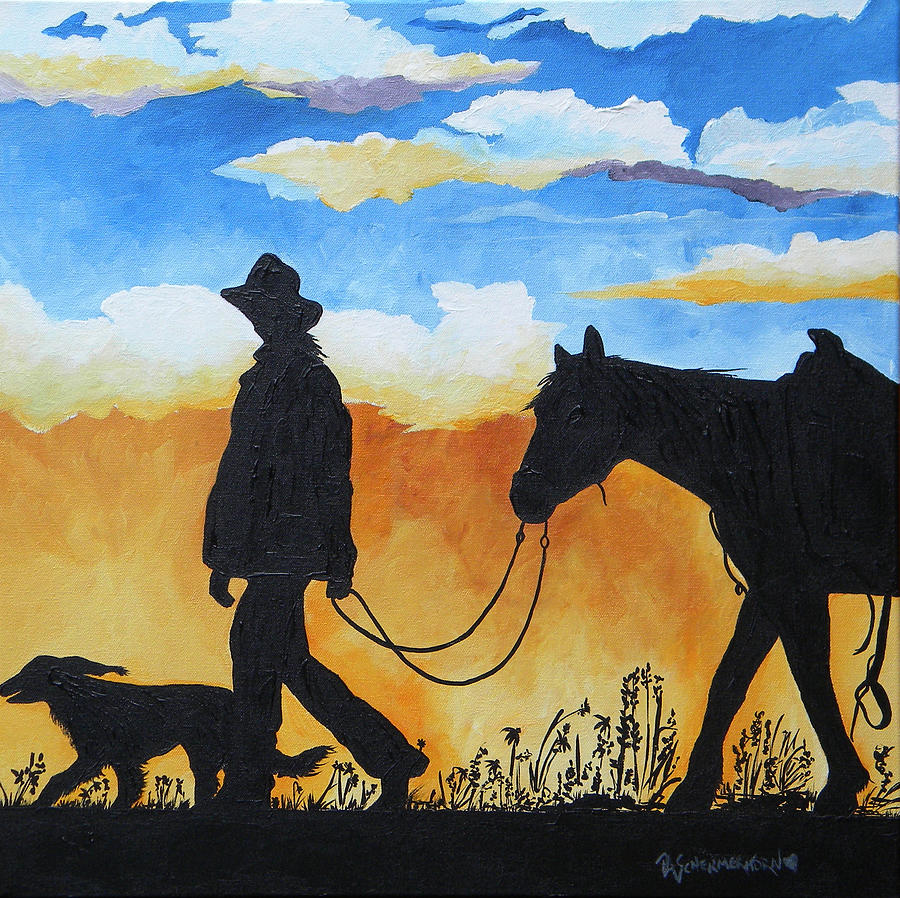In this evocative painting, the viewer's focus is drawn to the silhouettes of a cowboy or cowgirl, a horse, and a dog, all in shadow, against a vibrant and contrasting background. The central figure, a slender woman adorned with a cowboy hat, is leading the horse by its reins. The dark outlines of her form, the horse, and the dog are subtly highlighted with touches of white, hinting at their shapes without giving away intricate details. The scene is set in motion, with the trio walking to the left across a darkened ground dotted with small wildflowers and grasses.

Above them, the sky is a stunning gradient, starting with an orange glow near the horizon that transitions through shades of gold, purple, and white, finally merging into a brilliant blue at the top. Horizontal clouds streak the sky, adding depth and complexity to the scene. The bold contrast between the black silhouettes and the luminous sky enhances the painting's dramatic effect.

In the bottom right-hand corner, there is a signature in cursive that might read "Cher-Me-Horn," marked with a small heart, adding a personal touch from the artist. This painting beautifully captures the simplicity and quiet majesty of a moment at dusk or dawn, with its striking play of colors and shadows.